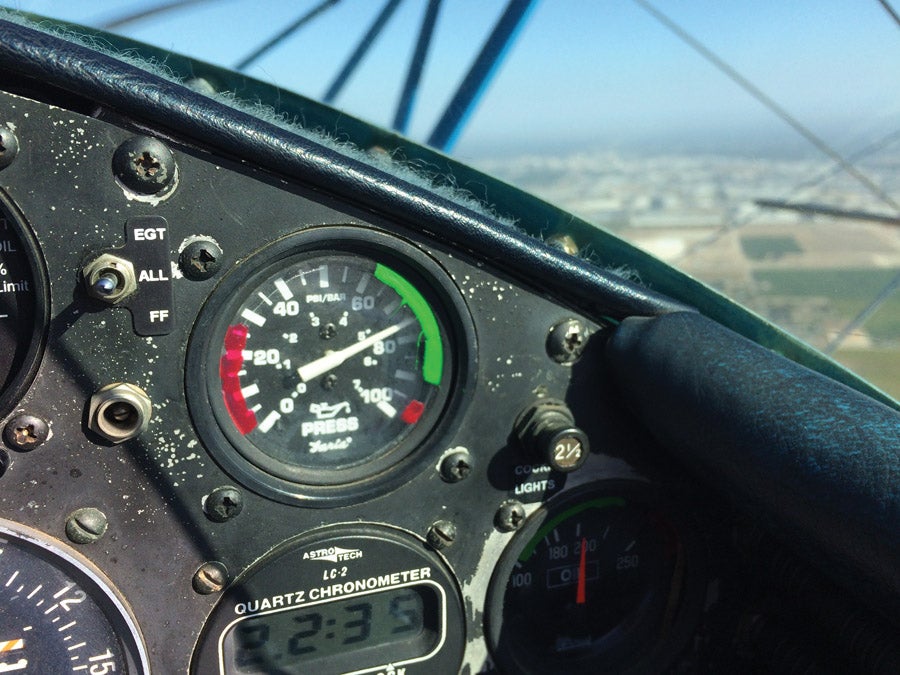The photo captures the cockpit of an older open cockpit or possibly biplane aircraft, indicative by the visible bars or wires crossing the image. The instrument panel, located on the right side of the photo, is partially illuminated by sunlight, creating a glare on the metal surfaces where paint is flaking off. This wear aligns with the age of the plane, though it features newer instruments. Prominently displayed is a gauge with a dial measuring from 0 to 100, currently positioned just under 80. Beneath this gauge is a digital quartz chronometer displaying time, possibly reading 2:35. The upper right corner of the image reveals a view down to the ground, showcasing buildings and a patchwork of green and brown fields. Various screws, buttons, and other instruments are scattered throughout the panel, contributing to the detail and complexity of the cockpit.